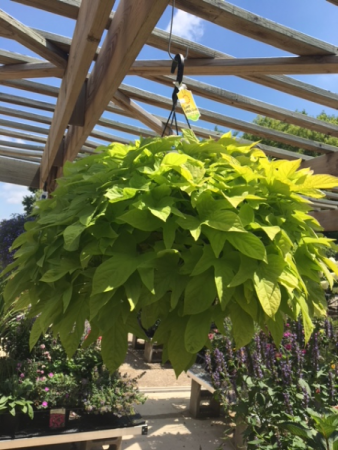The image showcases a very large, leafy plant hanging from the rafters of an open-air greenhouse. The plant, approximately two feet in diameter, has an abundant array of light green leaves that completely obscure any view of its pot. It is suspended by a plastic hook, which also features a tag. The hook is attached to a thin metal bar connected to sturdy wooden beams forming the ceiling. The background reveals numerous other plants, including small purple and pink ones, creating a lush, varied scene. The ground below consists of a mix of concrete walkways and gravel, flanked by wooden benches that support more plants. The scene is illuminated by an open blue sky with scattered clouds, giving the space an airy, expansive feel. Overall, the detailed, leafy plant is the focal point amidst a vibrant, well-organized greenhouse setting.